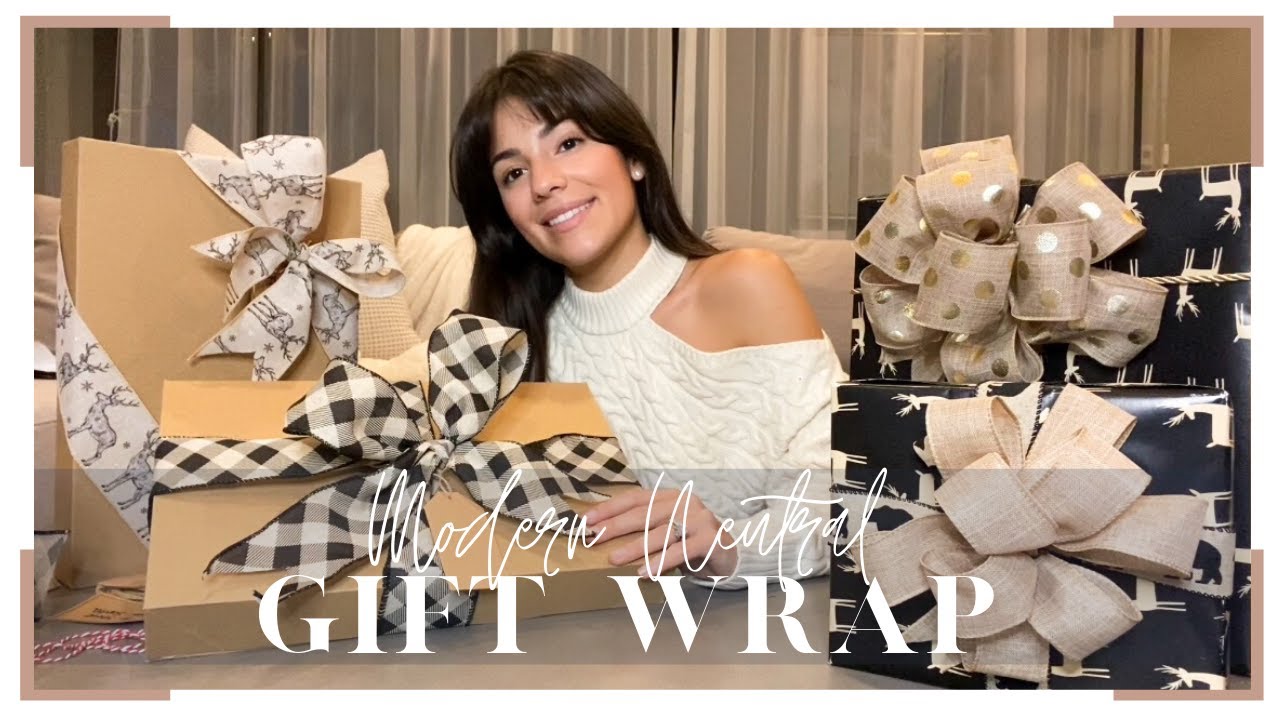In the photograph, a young woman with dark brown hair and bangs, wearing a stylish white turtleneck sweater with braided design and cut-out shoulders, poses and smiles at the camera. She sits on a tan sofa, with a beige curtain featuring a folded design in the background. In her left hand, she holds a rectangular cardboard gift box adorned with a plaid bow. Surrounding her on the table in front of her are several other gift boxes: to her left, two gold-colored rectangular boxes wrapped with black and white ribbons; to her right, two large rectangular boxes wrapped in black paper with white reindeer designs, tied with beige and burlap bows accented with golden polka dots. At the bottom of the image, in transparent and bold white font, the text reads "modern neutral" followed by "gift wrap." The scene exudes a festive and elegant atmosphere, emphasized by the neutral tones and modern gift-wrapping styles.